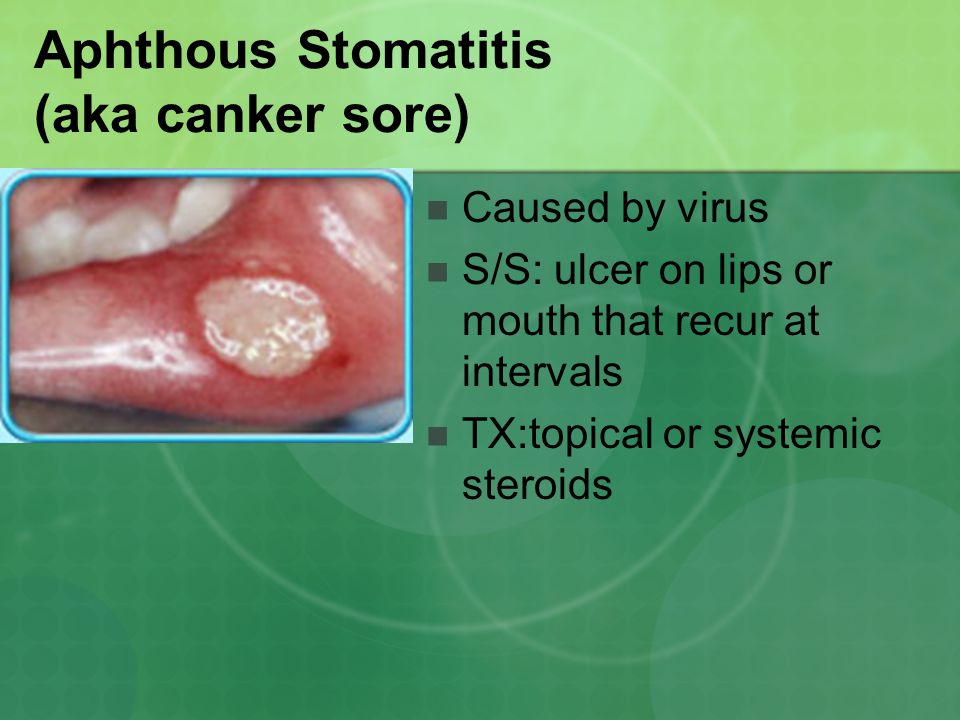The image is a detailed slide likely from a presentation, such as a PowerPoint or a website about canker sores, medically known as aphthous stomatitis. The slide is divided into two sections: a light green top section and a larger dark green bottom section. In the upper left corner of the light green section, bold black text reads "APHATHOUS STOMATITIS," followed by the explanation "(AKA canker sore)" in parentheses. 

The dark green section contains a rectangular photo in the upper left area, bordered in blue, showing a canker sore on a lip, with three teeth visible next to the sore. To the right of the image, there are three bullet points in gray with black text: 
1. "Caused by virus."
2. "S/S: Ulcer on lips or mouth that recur at intervals."
3. "Tx: Topical or systemic steroids."

The background features faint white circles, some colored in with the same light and dark green shades.